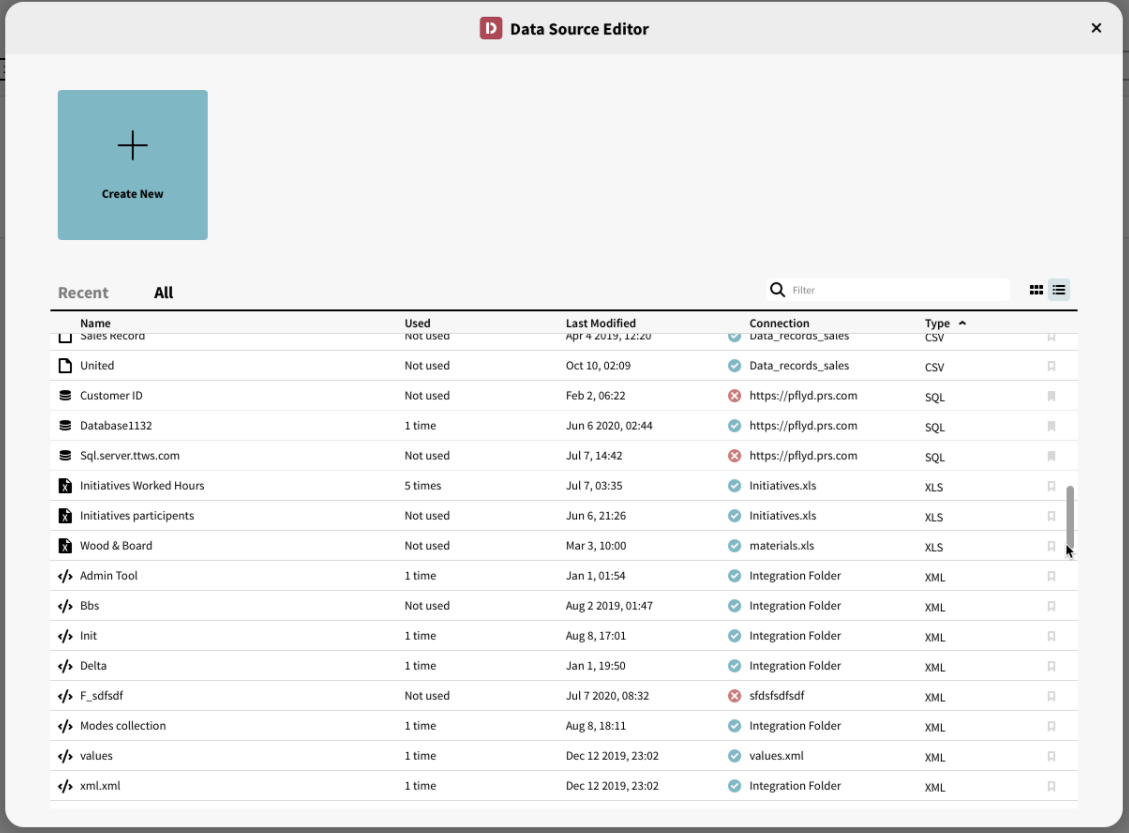This image is a screenshot of an interface titled "Data Source Editor," featuring a prominent logo of a red cube with a white letter "D." The primary background is a light gray tone. Central to the image is a large blue square, approximately one inch by one inch, containing a black plus sign and the text "Create New" in black font with initial capitalization.

Below this central element are several tabs labeled "Recent" and "All," accompanied by a search icon and a filter option. This section allows users to toggle between different views and search through data. A horizontal line separates this upper section from the detailed listings below.

In the lower section, a table is organized into columns with headings "Name," "Used," "Last Modified," "Connection," and "Type." These columns appear to contain information about various files, including their usage status, modification dates, connection details, and file types. The interface likely allows sorting by these columns, enabling efficient data management.